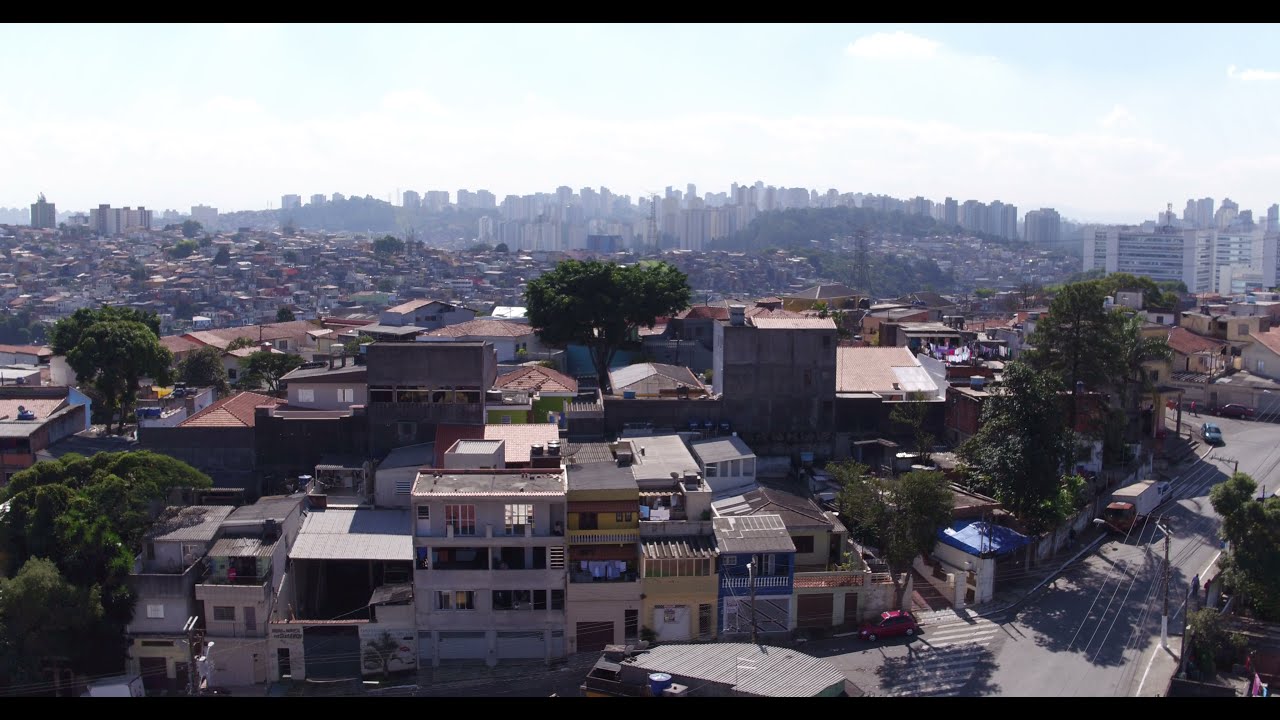This is a horizontal rectangular aerial photograph of a densely populated urban area, most likely a city in South America, potentially in Brazil judging by the dense build-up that resembles favelas. In the foreground, there are various buildings that could be apartments or houses, situated very close together, creating a crowded appearance. A street with cars and pockets of trees can be seen interspersed among the buildings. Towards the middle of the image, there are taller buildings that could be different types of residential structures or small apartment complexes. The landscape appears hilly with houses stretching out on the left side, and a more grassy area on the right, adding a sense of topography to the urban sprawl. Further back, there is a notable park area leading up to a cluster of industrial-looking buildings. Along the horizon, an array of towering gray skyscrapers forms a discernible skyline, though the individual structures are indistinct due to the overcast, grayish-blue sky that adds a muted tone to the entire scene. The overall impression is of a bustling, high-density cityscape, marked by a mix of architectural styles and urban elements.